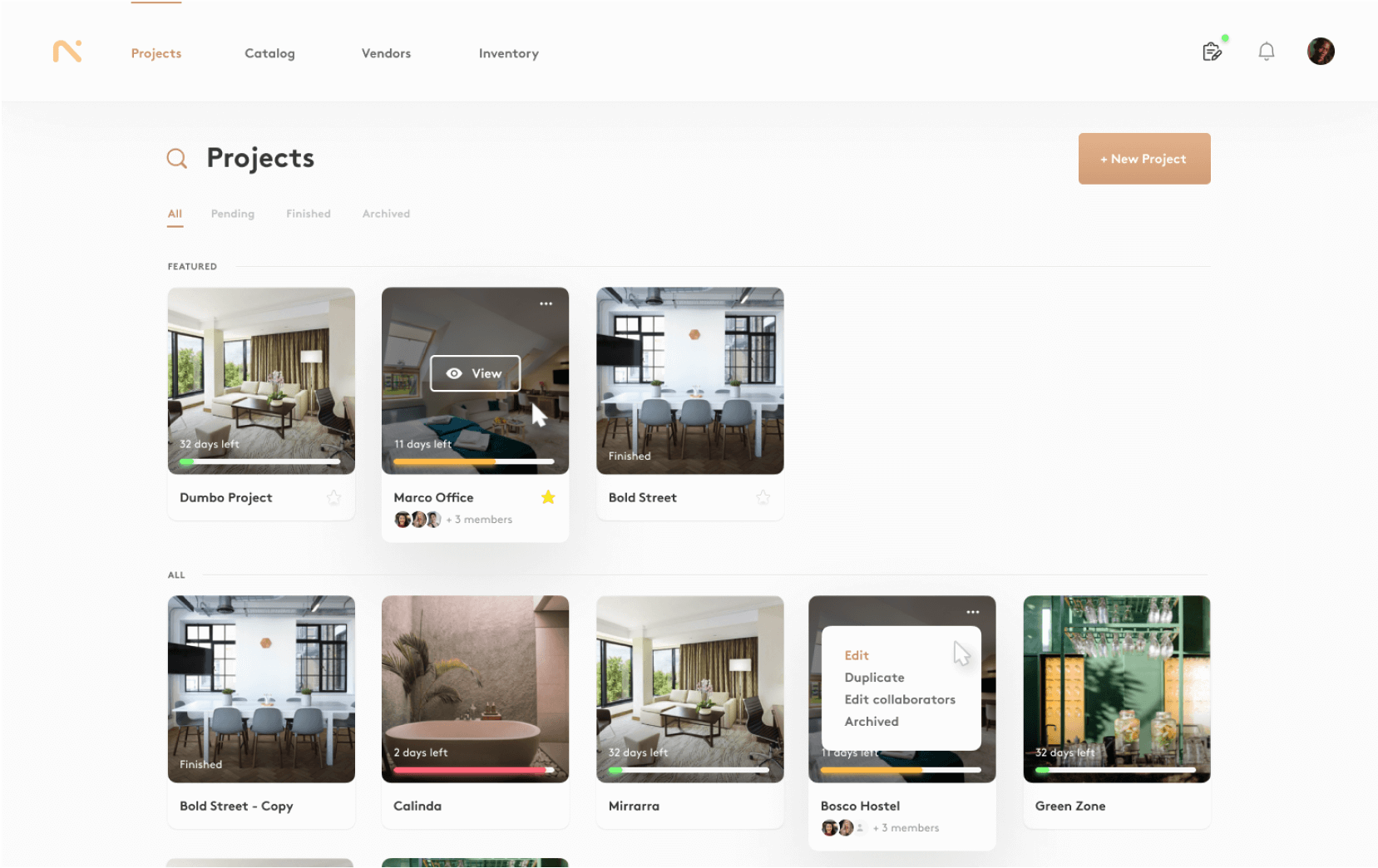The screenshot captures a website interface with a focus on project management. In the top-left corner, there is a distinct logo resembling an upside-down 'V' slanting diagonally towards the bottom right. Adjacent to the logo is the navigation menu featuring several tabs: "Projects," "Catalog," "Vendors," and "Inventory." The "Projects" tab is currently active, highlighted in orange, indicating the user is on the Projects page.

Directly below the navigation bar, the word "Projects" is displayed in bold black text, accompanied by a search icon to its left, facilitating quick searches within the projects section. On the far right of this section, there is a prominent pale orange button labeled "+ New Projects," allowing users to initiate new projects with a simple click.

In the top-right corner of the interface, there are several user tools, including a profile picture, a notification bell, and an icon resembling a notepad or a checklist, marked by a green dot at its top-right corner, possibly denoting some alert or status.

Under the "Projects" heading, categories like "All," "Pending," "Finished," and "Archived" are listed, helping users to filter their projects accordingly. The interface also displays specific project tabs such as "Featured," "Dumbo Project," "Marco Office," and "Bold Street," presenting an organized view of ongoing and highlighted projects.